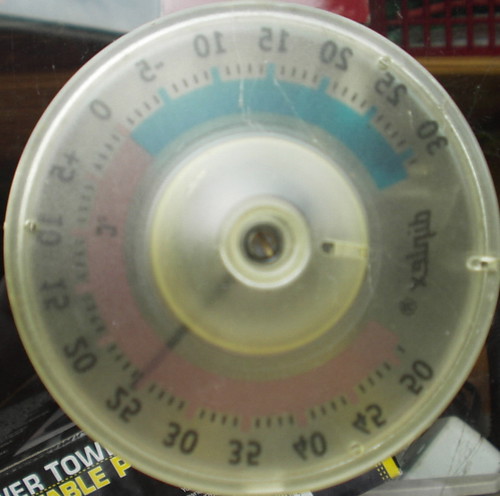The image features a somewhat vintage-looking device that appears to be a thermometer or possibly a timer. The device has a large, well-worn circular plastic top, suggesting it is not brand new and might date back to the 1980s. The face of the device is marked with a range of numbers, starting from 50 at the top and descending to zero. The scale features a gradient design with pink on one side and aqua blue towards the top, which likely indicates temperature ranges.

At the center of the circular face, a black needle points outward, presumably indicating the current temperature or time. The background of the image is indistinct, but there is a hint of a possible wooden floor in the upper left corner. On the lower left, part of a box is visible with partially obscured text. The visible part of the text reads "town,” with the upper half of the text in white and the lower half in yellow. The overall context of the setting remains unclear due to the lack of detailed background elements.